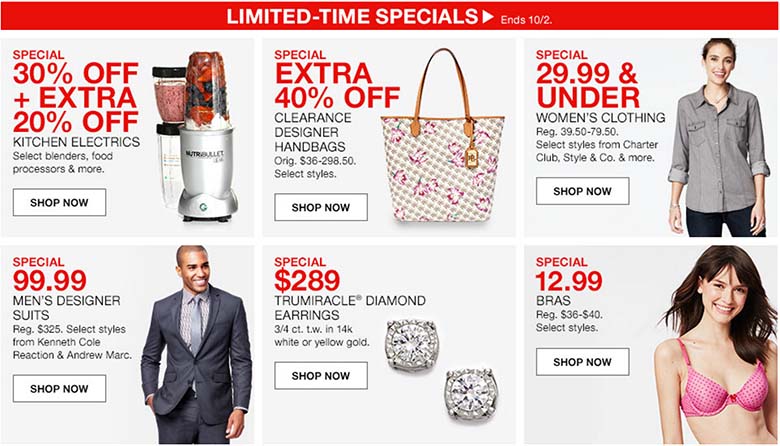The image showcases a promotional flyer for a store's limited-time specials, featuring various items on discounted prices, all displayed against a red background. At the top, bold text announces "Limited Time Specials," with the offer ending on October 2nd. Below this header, the layout is divided into six distinct sections, each highlighting different products.

1. **Kitchen Electronics:** On the left, the flyer advertises "Special Extra 30% Off, plus an additional 20% off" on select kitchen electronics including blenders and food processors. The section features images of two different blenders. A "Shop Now" button is available for immediate purchasing.

2. **Designer Handbags:** The central section promotes "Special Extra 40% Off" on clearance designer handbags, originally priced from $36 to $298.50. The example displayed is a designer handbag adorned with floral prints. The "Shop Now" button is prominently placed for convenience.

3. **Women's Clothing:** This offer includes "Special $29.99 and Under," on women's clothing that typically ranges from $39.50 to $79.50, featuring brands like Charter Club and Style & Co. The image shows a light-skinned woman wearing a pocketed, button-down shirt with rolled-up sleeves, paired with black pants.

4. **Bras:** The section advertises "Special $12.99" on select styles of bras regularly priced between $36 and $40. Illustrated is a woman modeling a pink bra. As with other products, a "Shop Now" button is available.

5. **Diamond Earrings:** In the center, a "Special $289" offer is highlighted for Triumviracle diamond earrings of 3-4 CT-TW, available in 14K white or yellow gold. Image showcases a pair of diamond earrings, accompanied by a "Shop Now" button.

6. **Men's Designer Suits:** On the far right, the flyer promotes "Special $99.99" on men's designer suits that are originally priced at $325. Featured brands include Kenneth Cole Reaction and Andrew Marc. The example image shows a smiling, dark-skinned man wearing a gray suit and tie.

Each section is aesthetically arranged with relevant imagery and price details to attract prospective buyers, further emphasized by the consistent presence of a "Shop Now" button for quick access to the store's online purchasing platform.